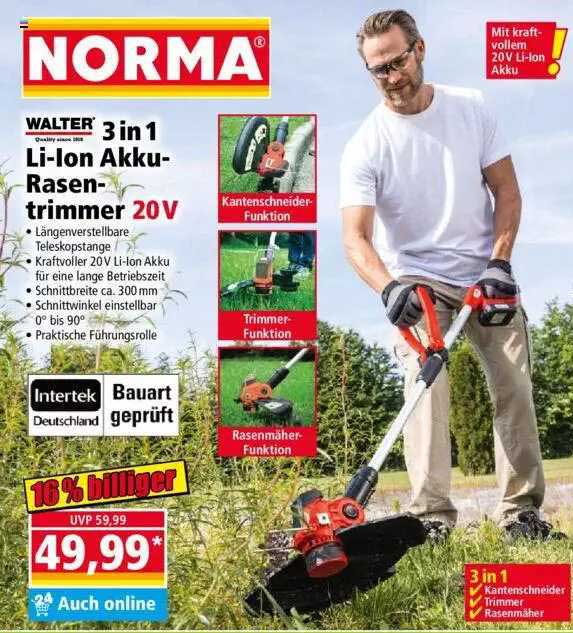The image is a detailed advertisement poster showcasing a man operating a trimmer on the grass. The man, a white male with blonde hair, is attired in a white t-shirt, khaki pants, and clear safety glasses, complemented by working gloves. He is depicted cutting through weeds with a battery-powered weed whacker, which features an orange handle, a silver post, and a black cutting base. The background captures a bright blue sky and lush green trees enhancing the outdoor setting.

On the left side of the poster, the brand name "LORMA" is prominently displayed in white lettering on a red rectangle with yellow trim. Below the logo, there are several lines of text in a foreign language, presumed to be German, that describe the product as a "three in one" Lian Aku Raisin Trimmer, 20V. The poster also includes smaller images showcasing the weed whacker's various functions.

Further down, the advertisement mentions "Intertec Dutchland" and "Bowerd Grapefruit," likely indicating additional features or specifications. A noted 16% discount brings the price down from 59.99 to 49.99, with the offer labeled "UVP." Additional text includes the phrases "24 odd or 9" and "three in one Cantor's Trimmer Resemper" near the bottom right of the poster. The scene and layout effectively highlight the product's utility in a visually engaging manner.